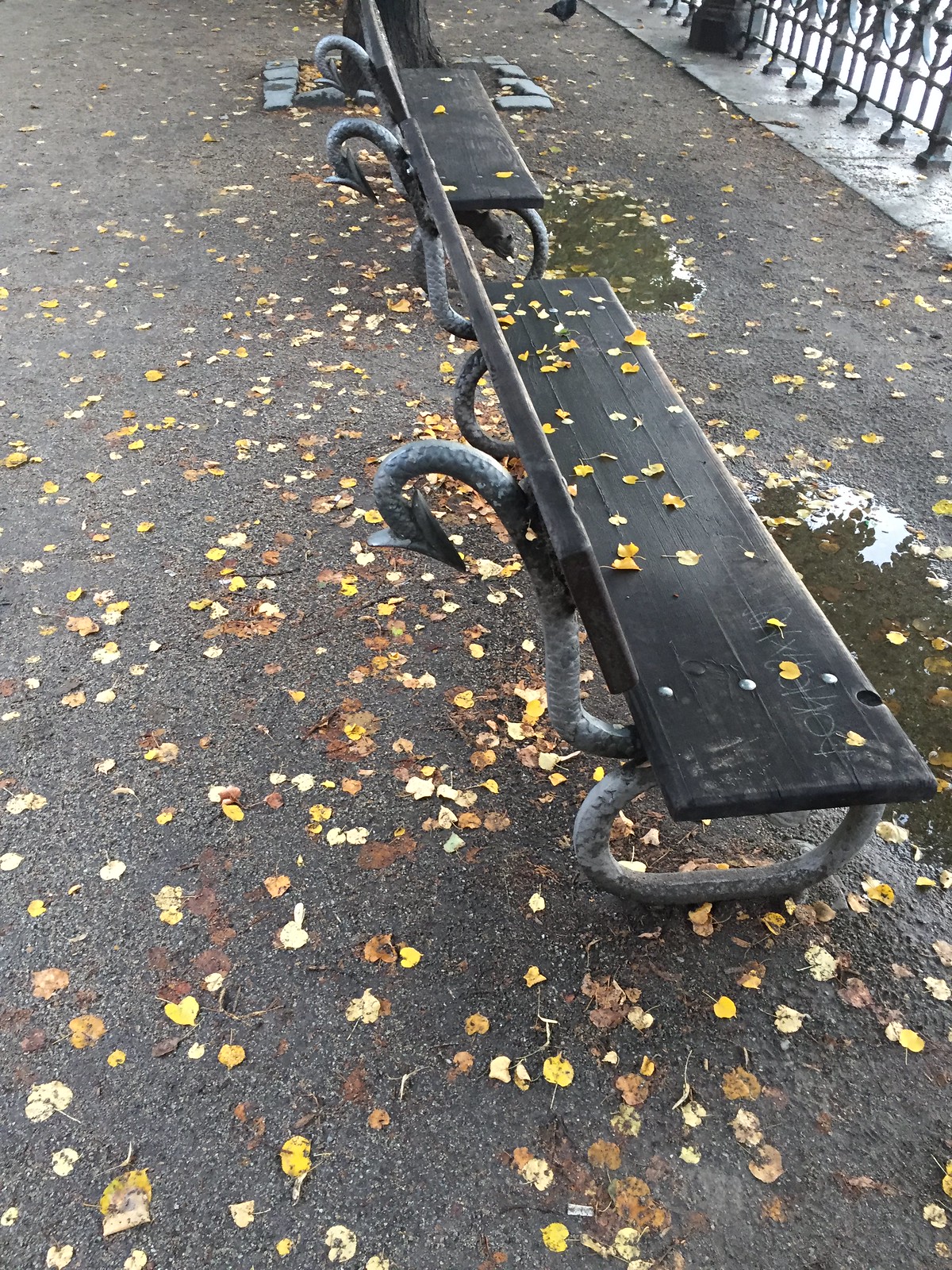This detailed photograph captures a park scene on a cloudy, fall day, with the ground all around wet and littered with yellow and brown leaves. Two prominent park benches made of dark gray wood and weathered, stylized metal frames resembling dragon tails with scales and spiky tips are set on a muddy, dark gray concrete surface. These benches curve gently and extend from the lower right towards the top center of the image, forming a perspective that draws the eye. The ground in front of the benches features small puddles reflecting tree branches, enhancing the damp, chilly atmosphere. To the right, a black iron railing or fence suggests either water or a drop beyond. A small tree trunk surrounded by gray pavers is just behind the benches, adding to the autumnal and serene park setting. The subtle detail of a bird, possibly a pigeon, is noted near the top of the image. The lighting is dim and muted, contributing to the overall cold and wet ambiance of the scene.